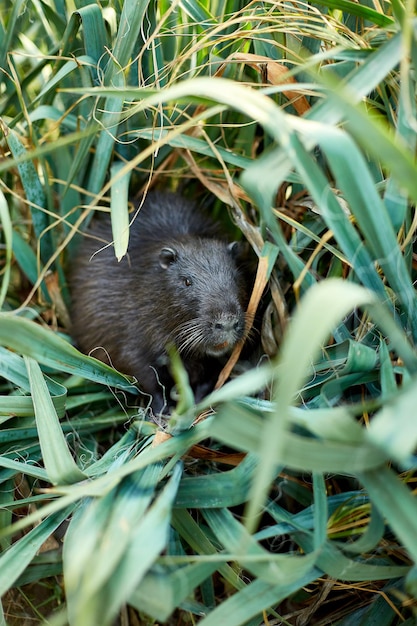In this detailed nature scene photograph, tall, thick green grass with occasional intermingling straw dominates the foreground, gently illuminated by a light source from above. Nestled among the long, slightly bent reeds and leaves, a small, furry mammal is the focal point. The animal, potentially a nutria or muskrat, features sleek, dark chestnut brown fur with small, bright black eyes. It has a broad head, a short, stout snout, and white whiskers. Rounded ears, slightly lighter in color and notched, protrude from its head. The creature's forelegs are visible and small, while its body appears plump with a thick neck. The animal is looking towards the camera, seemingly chewing on something, and exhibits a hint of orange teeth, suggesting it may be a nutria. The grass around it is a mix of green with occasional yellow and brown blades, adding contrast and depth to the scene. The sense of the animal hiding or being partially obscured by the grass enhances the photo's serene yet slightly mysterious atmosphere.